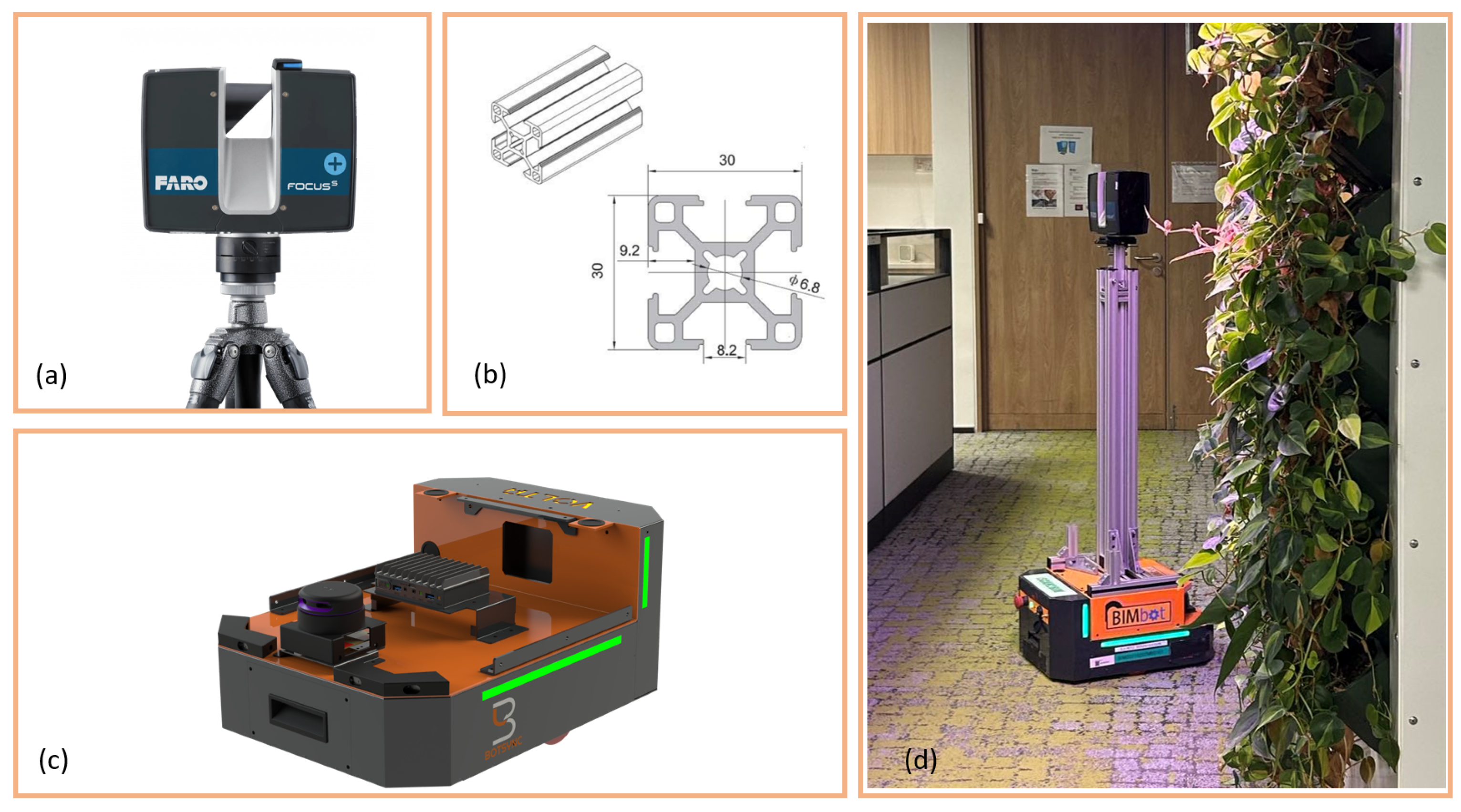This composite image showcases a detailed view of an industrial robotic device through four distinct frames labeled A, B, C, and D. 

Frame A, positioned in the top left corner, features a close-up of a grey and blue part of the device with the right side of the "Faro Focus" inscription visible. It is set against a white background. 

Frame B, located in the upper right, displays parts of the device that have been disassembled and measured, appearing in black and white. The measurements and schematic details of a bracket are clearly depicted, enhancing the technical precision of this frame.

Frame C, in the bottom left, shows what appears to be a charging station or stand, characterized by its grey and orange color scheme, situated on a white background. This frame gives the impression of a compact, functional piece of industrial equipment.

Frame D, the bottom right quadrant, presents the fully assembled device. The base of the device is prominently marked with "BIMBOT" on an orange background. The device itself has a black camera atop a tall grey pillar, resembling a camera on a tripod. The setting includes a textured floor, possibly vinyl or tile, surrounded by green ivy against a wall to the right, a brown double-door closet in the distance, and a lab-like counter with light brown cabinetry on the left. The backdrop adds context by including a kitchen cabinet visible in the top-left of the frame.

The overall composition effectively blends detailed schematic drawings and real-life photographs, offering an intricate look at the device from various perspectives and assembly stages.